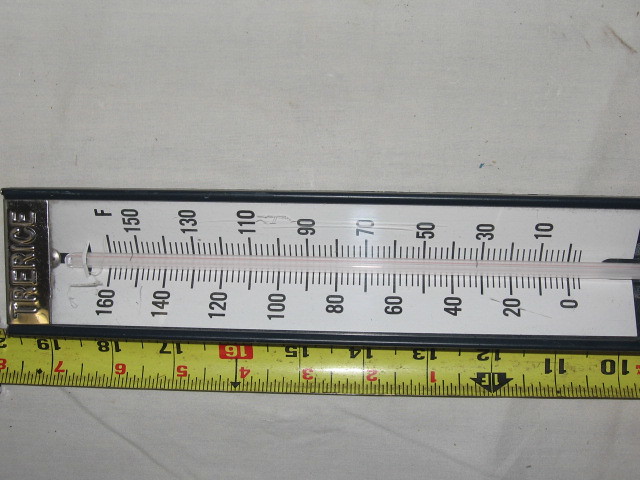This image features a wall-mounted thermometer, predominantly black around the edges with a white face and black lettering. The top portion of the thermometer is silver and it bears inscriptions that appear to spell "TRE" or "Tree Rice." Positioned beneath the thermometer is a yellow measuring tape with black and red numbers, indicating that someone is measuring the length of the thermometer. The scene is set on a table covered with a white cloth. The prominent colors in the image include white, black, yellow, red, and silver. The photograph meticulously captures the details and coloration of the thermometer and the measuring tape, highlighting the process of measurement.